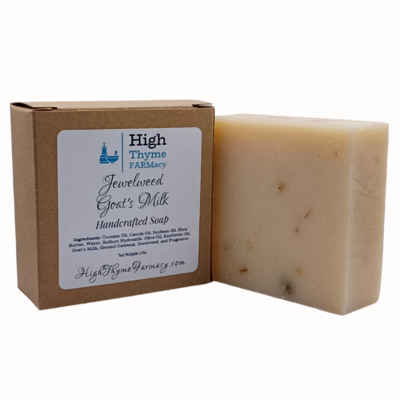This up-close photograph captures a rectangular bar of homemade soap and its packaging displayed to the left. The soap is predominantly beige with specks of brown interspersed throughout, and it features accents of yellow and orange at the top, giving it a handcrafted look. The soap appears substantial in size, suggesting it is a premium, artisanal product. The packaging is a plain brown box, adorned with a white label. The label prominently displays the brand name, "HI" in black text, followed by "TIME PHARMACY" in turquoise-blue text, and "JEWELWEED GOAT'S MILK HANDCRAFTED SOAP" in black text. The label also lists the soap's ingredients in very small, hard-to-read text, and provides the website "HIGHTIMEPHARMACY.COM" in cursive writing. Overall, the image conveys a sense of elegance and quality, highlighting the soap's natural and handcrafted qualities.